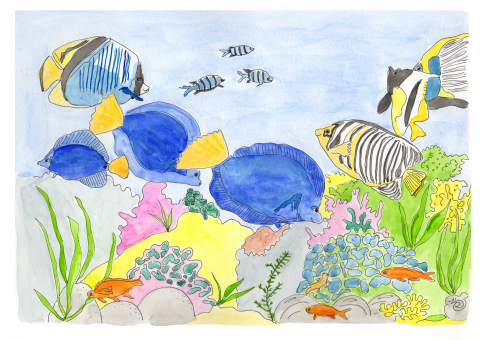The image vividly resembles a watercolor or colored pencil painting with a pastel palette, capturing a serene underwater scene of a coral reef. The background is painted in light blue, providing a tranquil backdrop for the vibrant, detailed coral at the bottom, which is depicted in shades of pink with green accents representing coral nodules and seagrass. A green patch with blue nodules contrasts with the coral, and there are a few yellow and darker pink blotches, as well as gray stones scattered around.

Above the coral, a variety of fish swim gracefully. The most prominent ones are flat fish with spiny fins extending from the crown of their heads to their tails. One fish is light blue with dark blue stripes and a yellow tail, while another is mostly white with black stripes and yellow accents. All the fish are depicted with small black dots for eyes. There are approximately six of these spiny-finned fish and three smaller blue fish with black stripes swimming together. The painting also features various other fish in different colors and patterns, including orange, brown, grey, and striped, adding to the rich diversity of the underwater ecosystem. The overall effect is a colorful, lively representation of marine life, as seen through the eyes of an imaginative artist.